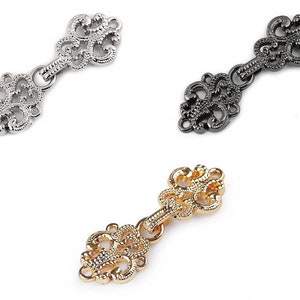This image features three ornate metallic pieces that appear to be jeweled accessories, possibly Victorian clasps or decorative elements for clothing or furniture. The items are arranged on a white background, diagonally upwards towards the right corner. Each piece showcases intricate artistic swirls and circles with a shape reminiscent of a fleur-de-lis on either side. The top left piece is a bright stainless steel silver, while the top right is a dark steely gray or pewter color, and the bottom one is a rich gold. Each has two connected parts, with the top part latched onto the bottom through a small circular clasp. Though they lack actual gemstones, the beading on these items reflects light similarly to diamonds, adding a touch of sparkle and elegance.